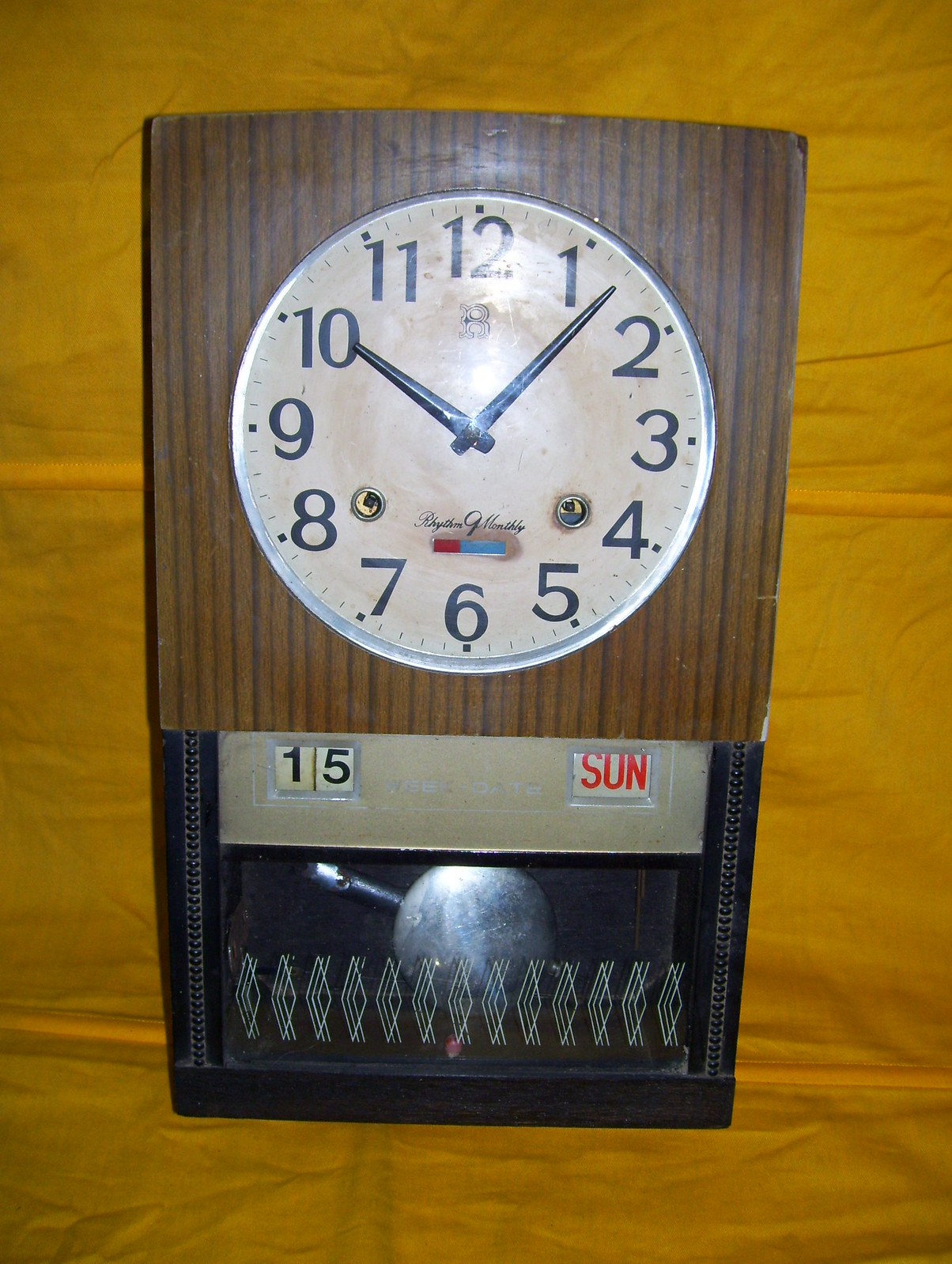A detailed photograph showcases a clock with a pristine white face, prominently positioned against a striped brown background. The clock face, meticulously numbered from 1 to 12, includes four small dashes between each numeral for precise time indication. Additionally, the face features two small circular holes, one situated next to the number 8 and the other next to the number 4.

In the bottom left corner of the image, the number "15" is printed in black, while the bottom right corner displays the word "sun" in striking red. Below the clock face, there is a shiny, silver round element with a horizontal bar extending to the left, appearing almost like a decorative pendulum. A piece of intricately designed glass, adorned with white diamond patterns, covers the clock face, adding a layer of elegance to the piece.

At the very base of the clock, a brown border with rivets on the right and left sides further emphasizes the timepiece's vintage aesthetic. Above the number 6 on the clock face, a blue and red line is visible, accompanied by small cursive writing that resembles "Raytheon."

The entirety of this sophisticated clock is set against a background that appears to be either tan wood or tan paper, enhancing the overall warm and classic feel of the image.